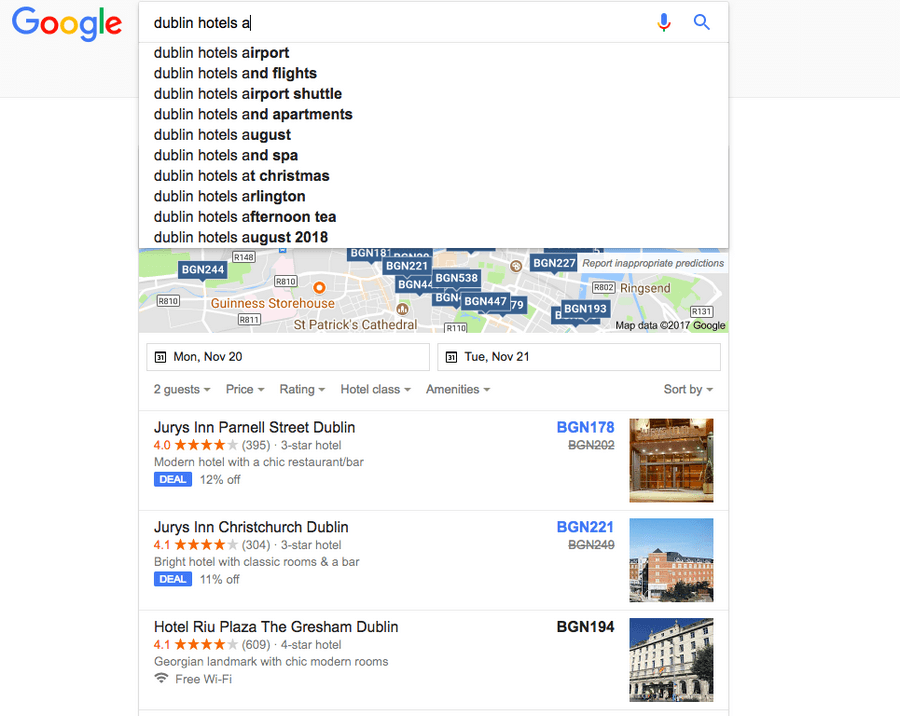The image depicts a screenshot of a web page featuring a search interface for Dublin hotels. At the top of the page, there is a gray banner. On the left side of this banner, the Google logo is displayed in its traditional rainbow colors, specifically blue, red, yellow, blue, green, and red. Below the banner is a search bar with a drop-down menu, initially filled with the text "Dublin Hotels A". The drop-down menu offers various suggestions, including:

- Dublin Hotels Airport
- Dublin Hotels and Flights
- Dublin Hotels Airport Shuttle
- Dublin Hotels and Apartments
- Dublin Hotels August
- Dublin Hotels and Spa
- Dublin Hotels at Christmas
- Dublin Hotels Arlington
- Dublin Hotels Afternoon Tea
- Dublin Hotels August 2018

At the top of the search bar are icons of a microphone and a magnifying glass. Beneath the search bar, there is a map displaying different streets, landmarks, and points of interest. Below the map, the dates "Monday, November 20th" and "Tuesday, November 21st" are shown, followed by filters for "two-guest price rating," "hotel class," and "amenities," each with drop-down options.

Further down, a list of hotel names is provided, including:
- Jurys Inn Parnell Street, Dublin
- Jurys Inn Christchurch, Dublin
- Hotel Riu Plaza The Gresham, Dublin